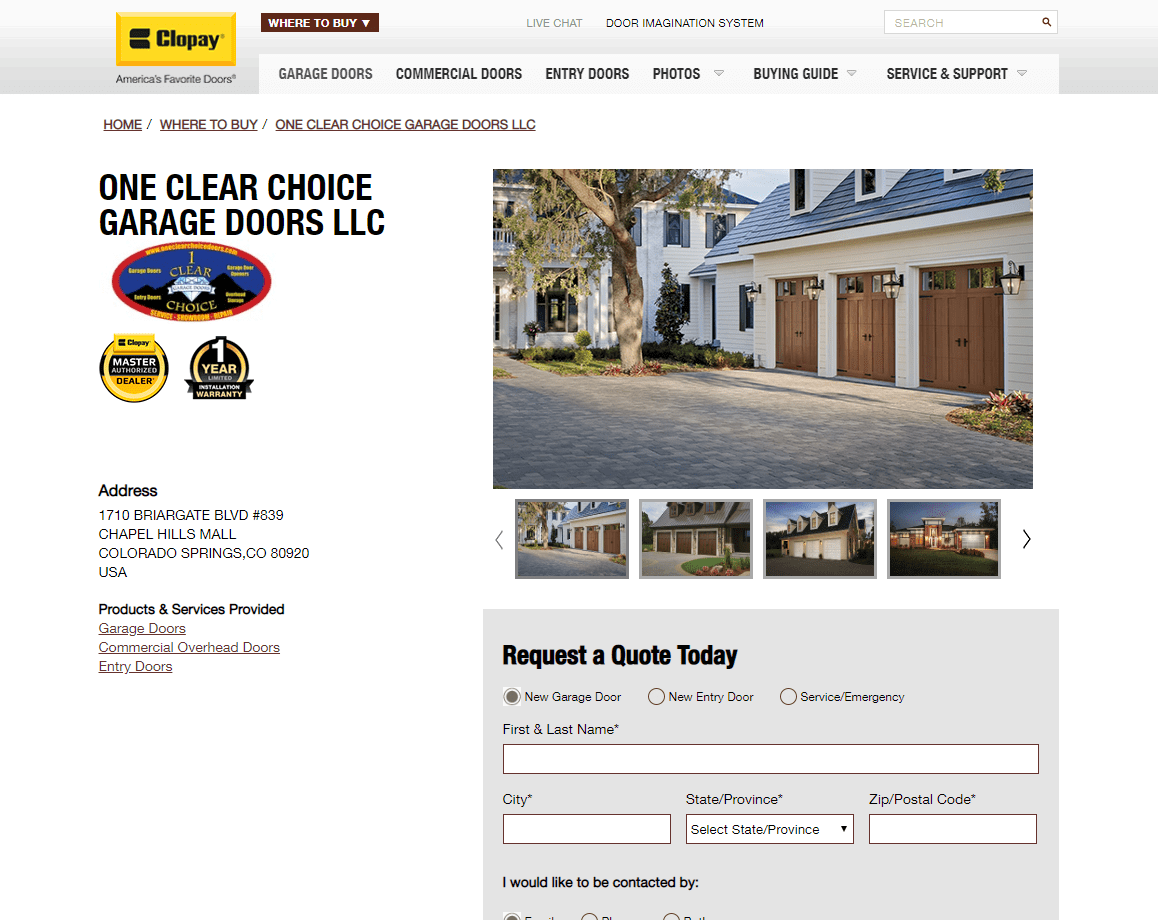The image features a detailed webpage layout for a garage door company. At the top, there's a grey background with a white button and black text spelling out "Coldplay" (C-L-O-P-A-Y). Below this, on a black background with white text, it says "This is where to buy them," accompanied by a dropdown menu. 

In the right center, in grey text, it states "This is live chat." Below this, in black text, it declares "This is door imagination system." On the right-hand side, there's a search bar.

Further down, towards the right, there's a white background with black text listing clickable buttons: "Garage Doors," "Commercial Doors," "Entry Doors," "Photos," "Buying Guides," and "Service and Support."

On the left-hand side, there is a thin black underlined text that reads "Home / Where to Buy / One Clear Choice Garage Doors, LLC," leading to a larger print of "Garage Doors, LLC." Below this are several photos, including one of a well-maintained house with tan and dark brown garage doors. Additional images feature white garage doors.

The company's address is listed as:
1710 Beargate Blvd, 
Number 839, 
Chapel Hill Mall, 
Colorado Springs, Colorado, 80920, USA.

The webpage also outlines the available products and services: "Garage Doors," "Commercial Overhead Doors," and "Entry Doors." 

Towards the bottom, there's a request form for a quote, asking for the user's first name, last name, city, state, and zip code.